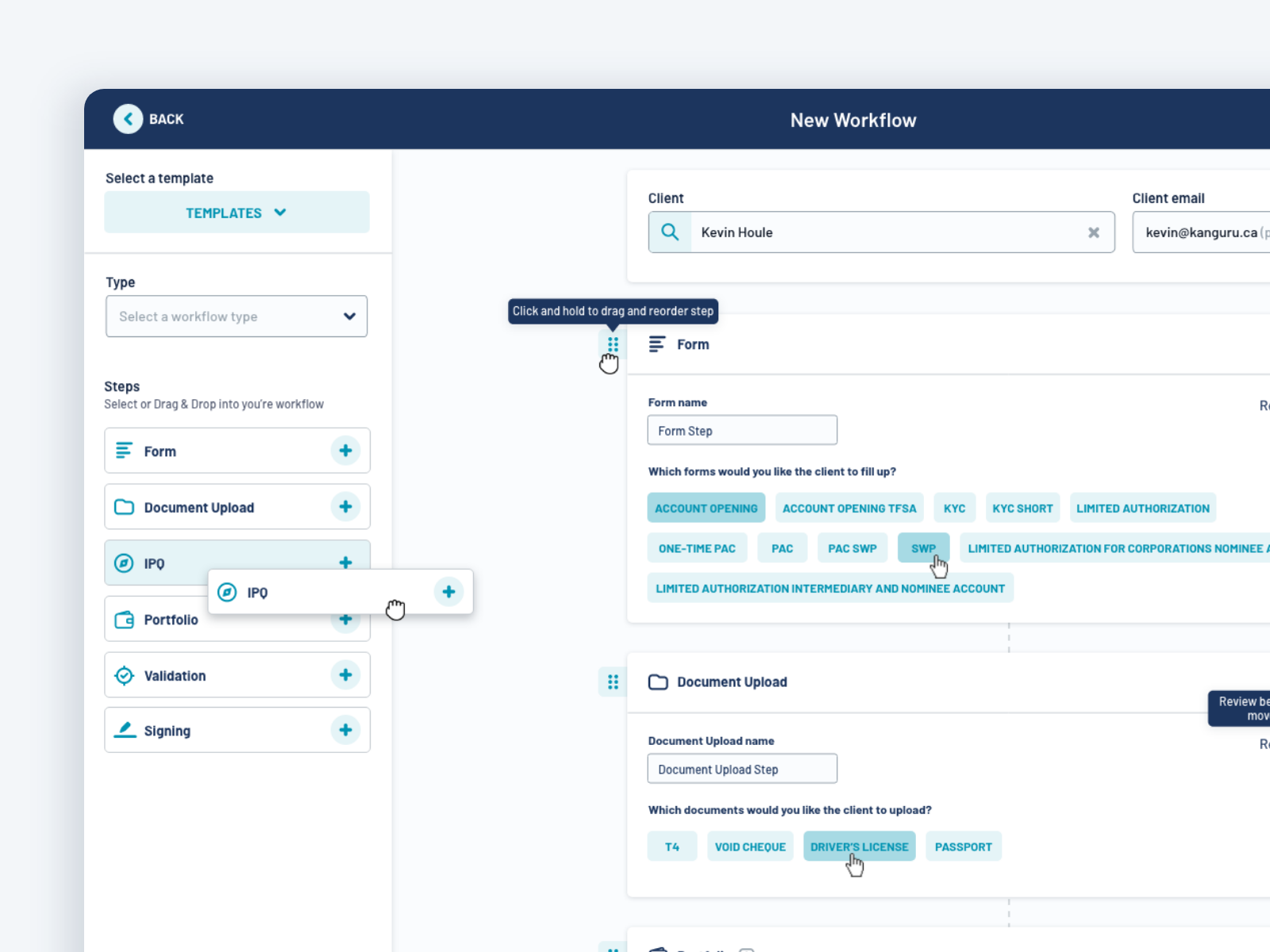In the screenshot, there is a detailed workflow interface displayed, comprising several steps for a client named Kevin Hill, whose contact email is kevin.kangaroo.ca. The workflow begins with an initial stage of dragging and dropping elements to formulate the process:

1. **Form + Folder**: This step involves uploading documents with elements that include:
    - **Document Upload**: Several documents like IPQs and portfolios need uploading. Each document type is indicated by a "plus sign."
    - **Validation & Signing**: This step ensures all submitted documents are validated and signed as needed.

2. **Form Configuration**: The next part of the workflow asks for form configuration:
    - **Client Details Display**: The interface sections display client details such as name and email at the top.

3. **Form Settings**: This includes setting up the form name and text for the form step, asking the user which forms the client needs to fill out:
    - Options include "Account Opening," "TFSA," "KYC," "KYC Short," "Limited Authorization," "One Time PAC," "PAC," "STVP," and specific types of limited authorization forms for nominees or corporations.

4. **Document Upload Configuration**: This step specifies which documents the client needs to upload, listing options such as:
    - Void check, driver's license, passport, and others.

The interface clearly allows for multiple elements to be dragged and dropped into the workflow to customize the client onboarding process efficiently.